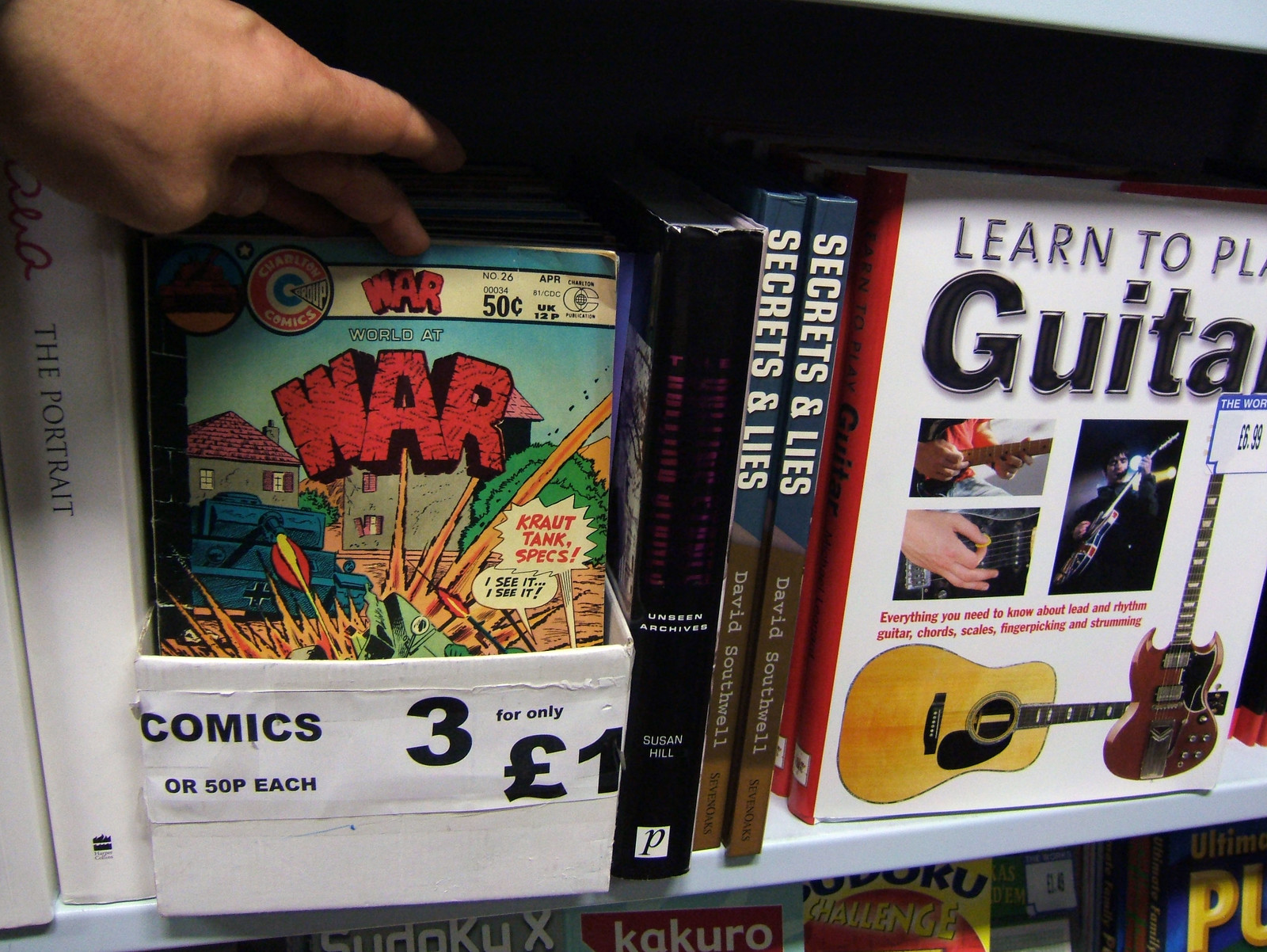In this image, we're looking at a close-up of a shelf in a store, specifically focusing on a section filled with books and comic books. The central focus is a white container labeled "COMICS," with a handwritten sign indicating prices: "50p each or three for only £1." A left hand, likely belonging to a Caucasian person, is reaching into the container to touch a comic book. This comic book prominently features the title "World at War," issue number 26, priced at 50 cents, with an illustration of an explosion and the words "Kraut Tank Specs" on the cover.

Surrounding the comic box, we see several books. On the left, a white spine reads "The Portrait." To the right of the comic box, a black binder's text is unclear, but next to it are two identical books titled "Secrets and Lies" by David Southwell. Facing outward is a book titled "Learn to Play Guitar," adorned with images of guitars. The shelf directly below shows more books, hinting at a variety of puzzle books with visible titles like "Sudoku Challenge" and "Kakuro."

Overall, the image conveys a cluttered yet intriguing view of a bookstore or a similar setting, with the main colors being white, black, red, and some yellow accents amidst the assortment of books and comics.